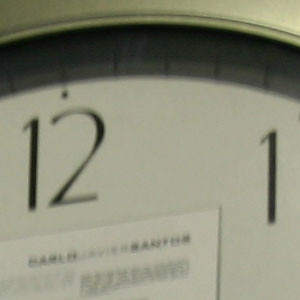The image captures a close-up of a clock's face, focusing on the section between the 12 and 1 o'clock marks. The black numerals stand out against a pristine white background, with three tick marks evenly spaced between each number. The entire clock face and its rim share the same white hue, blending seamlessly with the white backdrop on which the clock rests. In the bottom-left corner of the clock, a partially visible piece of paper lies where the clock hands would typically be, obscuring about 40% of the clock face. This paper features black text, though the text is blurred and illegible. The image also subtly highlights the shadow cast by an overhead light, which accentuates the clock's rim.